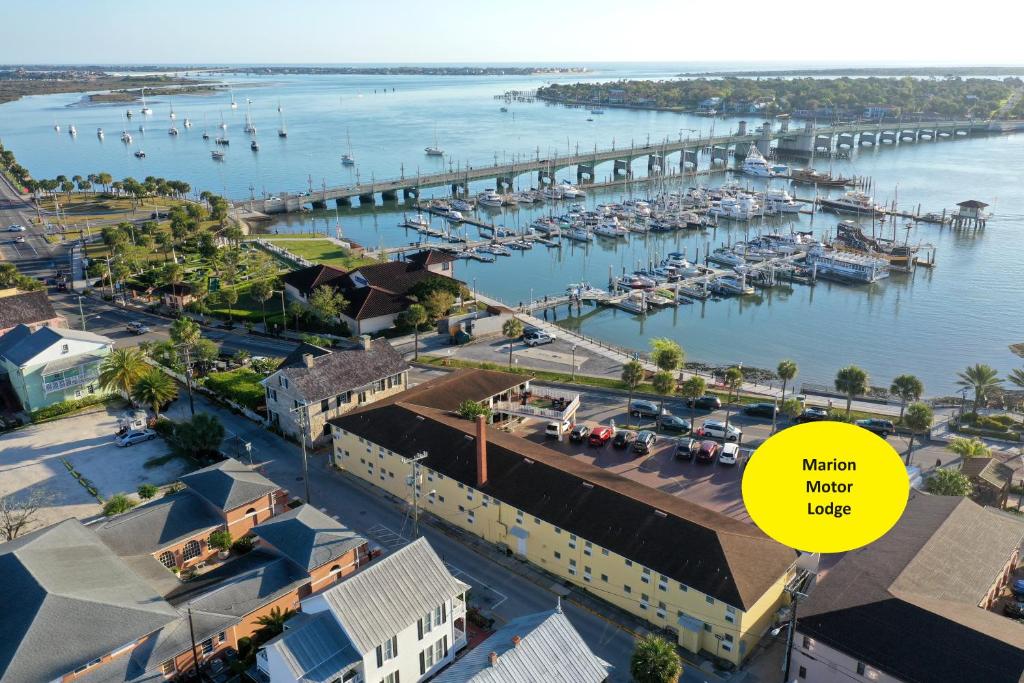The image presents an aerial view of a coastal area prominently featuring the Marion Motor Lodge, identifiable by a yellow circle in the lower right-hand corner of the picture. The lodge is a long, yellow building with a brown roof, situated next to a parking lot with about seven or eight cars. Adjacent to the lodge and its parking lot is a highway lined with a green strip and palm trees, and a wooden walkway is also visible nearby. The lower left corner of the image showcases the rooftops of some additional buildings and houses intermixed with streets.

Central to the image, two piers extend into a large open area of blue water, where numerous boats are docked. In the upper regions of the photo, a long bridge spans the water, connecting this area to another land section rich with trees, indicating a small town area. Scattered boats populate the water beyond the bridge. The scenery is soaked in daylight under a bright blue sky with the sun shining, encapsulating the vibrant atmosphere of the coastal town.